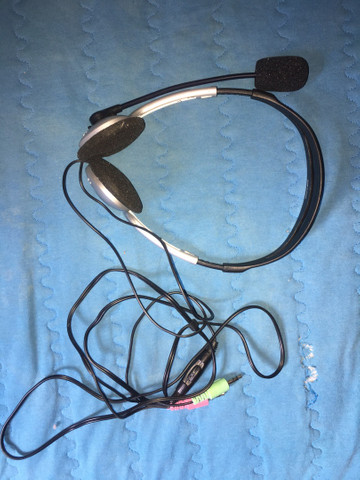This image is a color photograph in portrait orientation, featuring an old pair of headphones with a microphone, positioned prominently on a blue quilted fabric backdrop. The fabric background showcases intricate hand-stitched vertical zigzag rows, with noticeable wear where the stitching is coming apart at the bottom right corner. The headphones, centered in the upper portion of the image, sport a silver exterior with black ear discs and an adjustable black headband. Extending from one of the ear cups is a black stem holding a small black microphone. A black wire, originating from the bottom of the headphones, winds down gracefully towards the bottom edge of the image, ending in audio jacks—one yellow and one black—suggesting potential connectivity to various devices. The setting, potentially a bedroom or living room, provides a casual, lived-in feel to the composition. The scene is bathed in a spectrum of colors including blue, black, silver, green, pink, and white, capturing a moment of everyday realism.